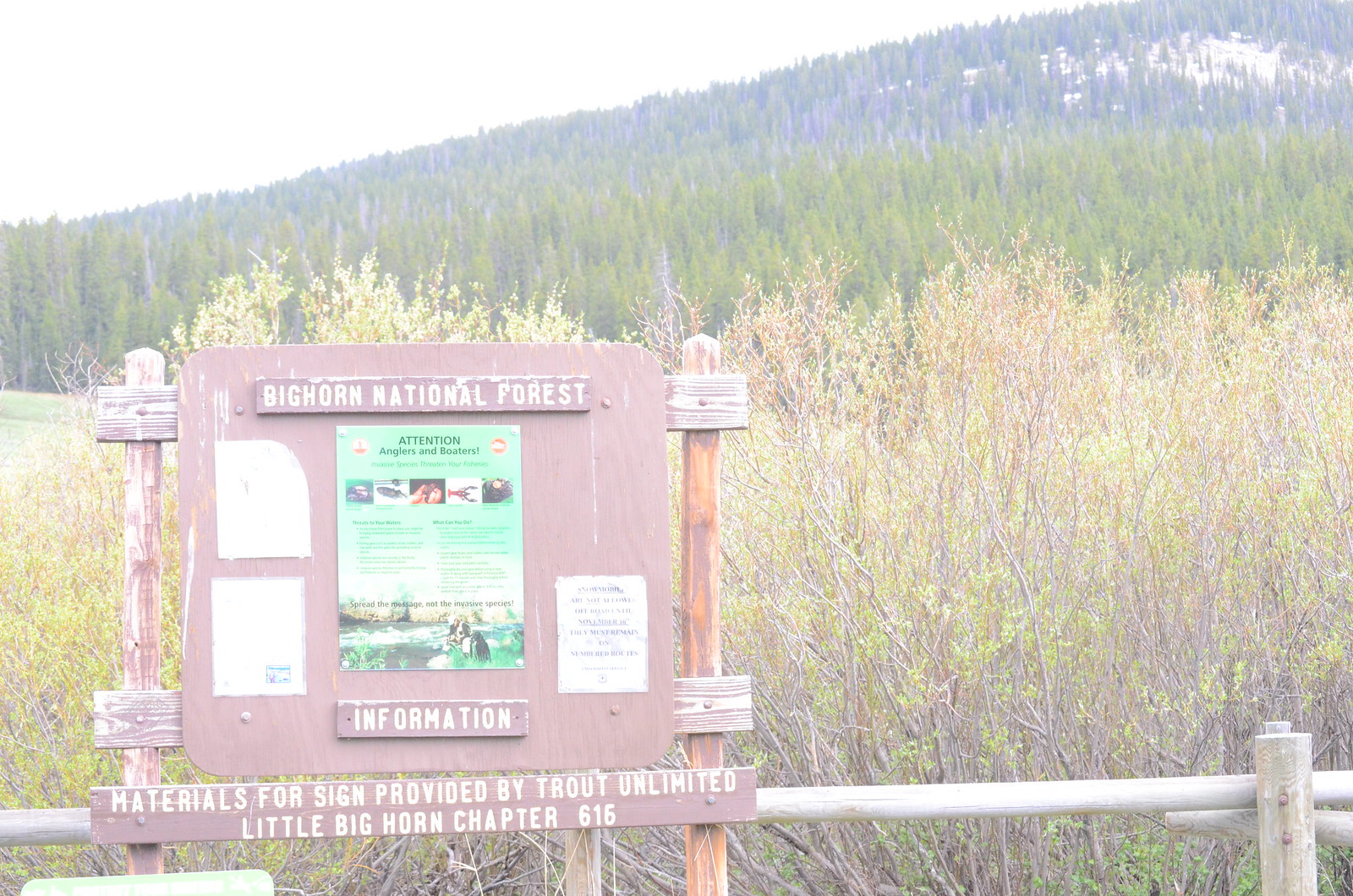The photograph, taken outdoors during the daytime, features a somewhat faded and muted quality. Dominating the lower left corner of the image is a wooden sign, purplish-pink in hue, bearing the text "Big Horn National Forest" in white print. Beneath this main text, the sign provides information, with a smaller, less legible section that reads "Attention Anglers and Boaters," followed by the difficult-to-read inscription, "Materials for sign provided by Trout Unlimited, Little Bighorn Chapter 616."

The foreground of the image shows a wooden fence, transitioning into various shades of tree cover. Closest to the camera are yellowish trees, giving way to a middle layer of darker green vegetation, and culminating in a backdrop of densely packed, deep green trees atop a mountainous terrain. In the upper left section of the photo, the sky appears grayish, hinting at overcast weather. This layered landscape of rolling hills, draped in a rich diversity of trees, stretches out towards the horizon, enhancing the natural beauty despite the subdued color palette.